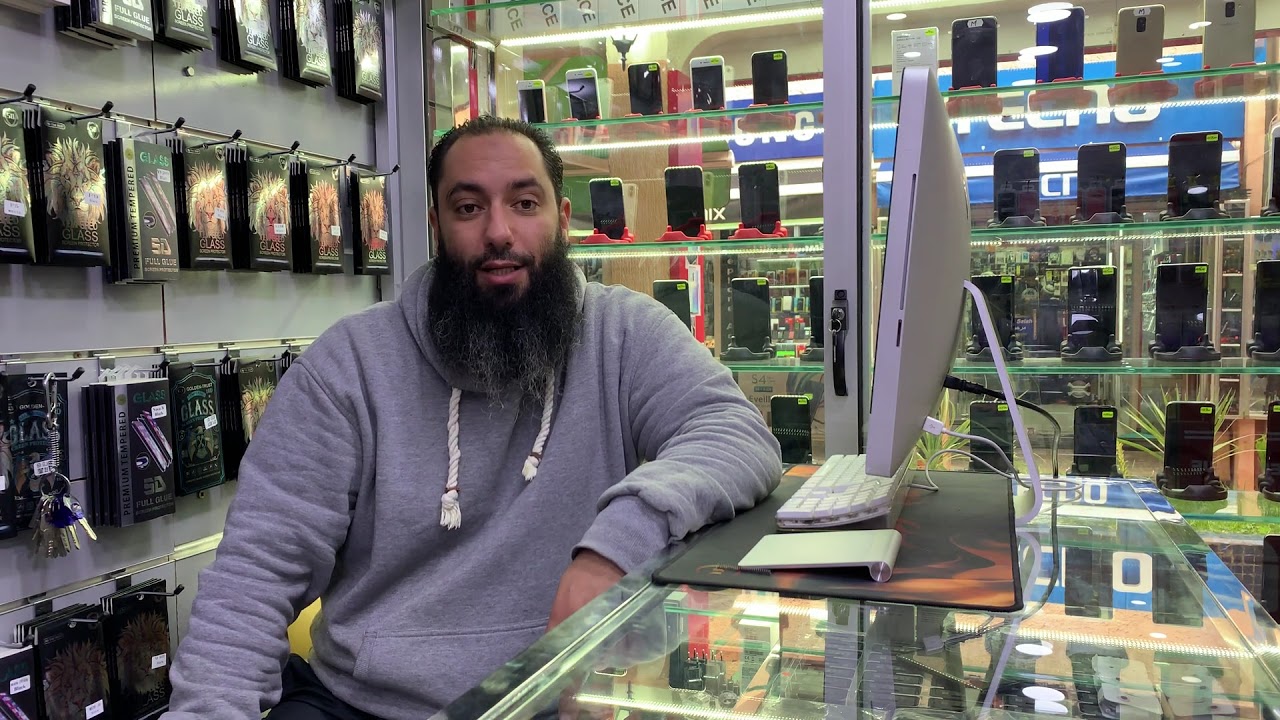In the photo, a bearded gentleman with dark hair and a mustache is seated behind a glass display counter in an electronics store specializing in smartphones. He is wearing a gray hoodie with white pull cords, and his arm is resting on the counter next to an iMac computer with a trackpad, which he is facing. The man appears to be engaged in conversation, as his mouth is slightly open, revealing his bottom row of teeth. Behind him, shelves filled with boxed merchandise, likely protective covers and accessories for smartphones, are visible. To the left of the image, additional shelves with games and other products are seen, with a key ring full of keys hanging on one of the pegs. The background reveals a transparent wall leading to an aisle, suggesting the store is located within a shopping mall.